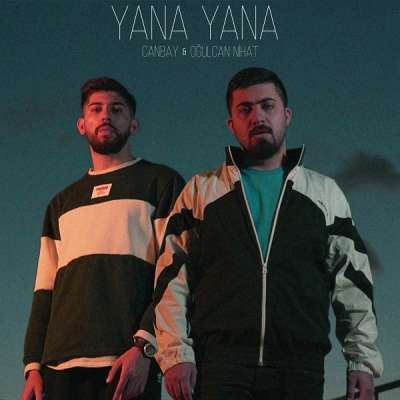Two men stand side-by-side at dusk against a dark blue background that lightens towards the bottom, accented by an overlay of tree leaves and white lettering at the top reading "YANA YANA" and "CANBE IN OGLAKENAT." The man on the right wears a partially unzipped, black and white jacket with white sleeves and two black bands on the arms, revealing a green shirt underneath. His dark hair is complemented by a beard and goatee, and his arms rest at his sides. The man on the left is clad in a long-sleeved shirt with wide black and white stripes—two black bands framing a central white stripe—and a white rectangular logo with indiscernible symbols near his collar. He has dark hair, a mustache, beard, goatee, and a watch on his left wrist, appearing to look downward. Both men wear black pants and have lighter skin tones, adding to the advertisement's cohesive visual presentation.